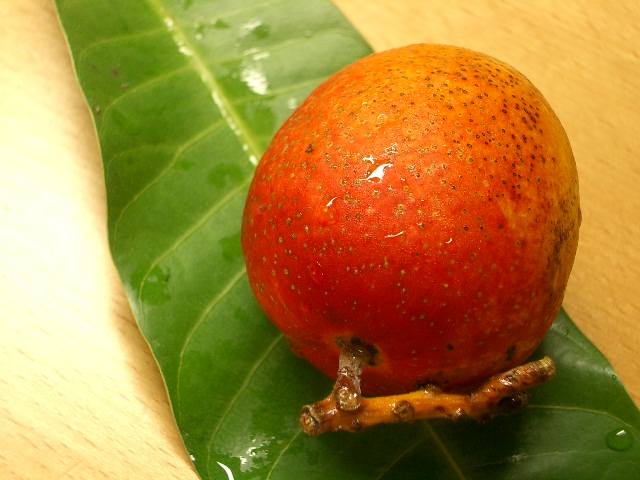In this photograph, a round, light orange fruit with darker orange and red hues is prominently displayed atop a large, green leaf that appears slightly wet. The fruit, which is likely tropical but not definitively identified, has a brown stem protruding from the top and its skin is spotted with brown discoloration. The leaf, possibly belonging to a large plant like a banana plant, is also wet and features a notable dewdrop on its bottom right edge. Both the fruit and the leaf rest on a light wood grain kitchen table, creating a natural, earthy setting. The entire scene suggests that the fruit might have been recently washed or exposed to rain.